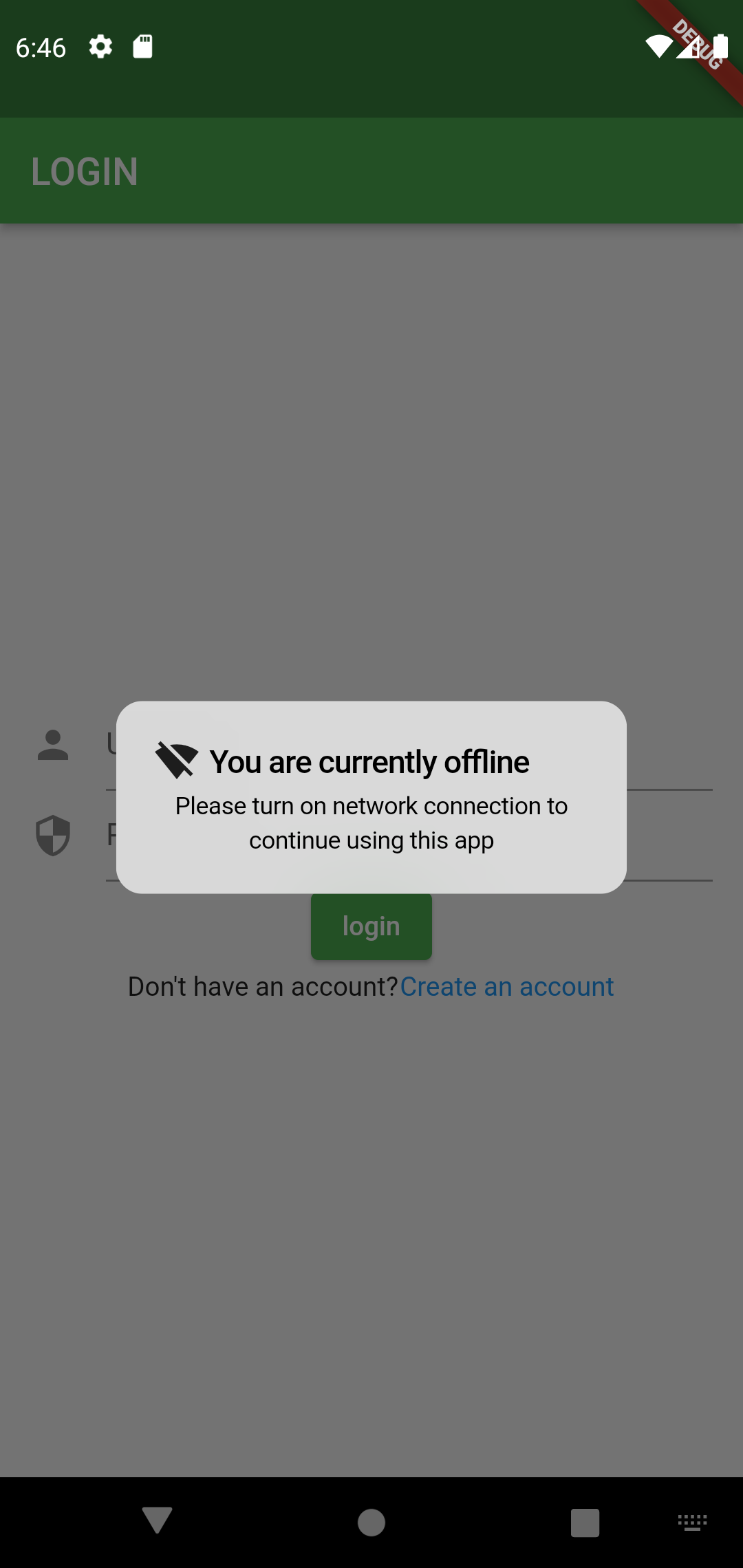This image is a detailed screenshot taken from a cell phone screen. At the very top, the time displayed is 6:46. On the top right corner, a red diagonal banner says "DEBUG" in bold white letters. The main screen has a grayscale overlay with a partially visible green button labeled "Log In." Superimposed over this main screen is a central pop-up window. This window features a Wi-Fi icon with a diagonal slash through it and a message that reads, "You are currently offline. Please turn on network connection to continue using this app."

Beneath the pop-up, part of the main screen is still visible, showing a green rectangle with the text "Log In" and a prompt that reads, "Don't have an account? Create an account." At the bottom of the screenshot, there are navigation icons including an arrow pointing down, a circle, a square, and what appears to be a keyboard icon. The image itself is portrait-oriented, meaning it is taller than it is wide. Notably, there are no photographic elements, people, animals, birds, plants, vehicles, airplanes, or helicopters in this image.